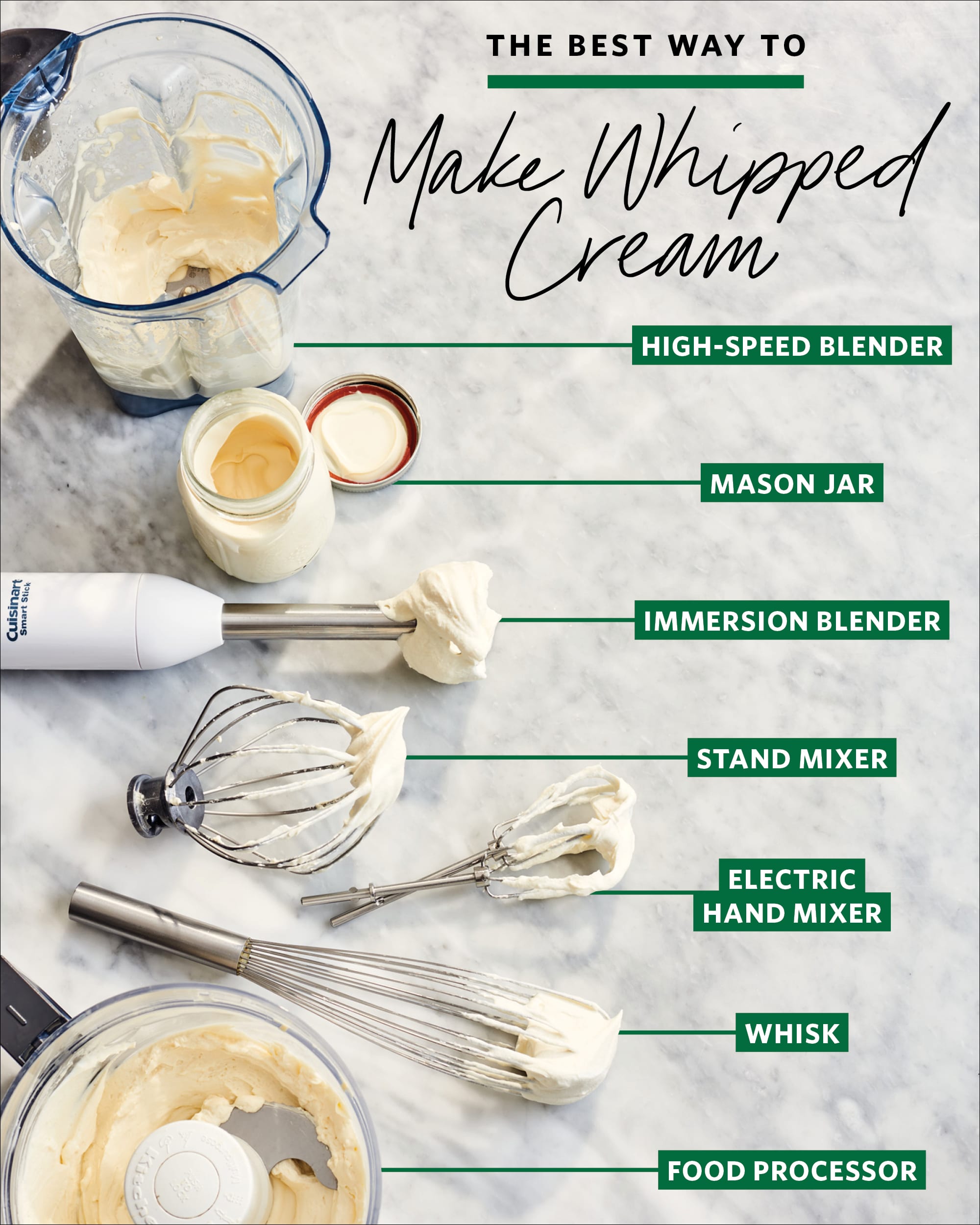The image is a highly detailed instructional guide titled "The Best Way to Make Whipped Cream," set against a gray, marble-like background. At the top, the title is divided into two distinct fonts: "The Best Way to" is written in bold black letters underlined by a green line, while "Make Whipped Cream" is in a cursive, fluid script. Down the left side of the image, there is an array of various kitchen implements, each with a label in a green rectangle containing white text. The implements, all smeared with whipped cream, include:

1. **High-Speed Blender**: Depicted with some remnants of whipped cream inside its pitcher.
2. **Mason Jar**: A clear jar filled with whipped cream, with its metal lid and seal placed nearby.
3. **Immersion Blender**: A white handheld mixer with a stainless steel shaft, showing whipped cream on its blending end.
4. **Stand Mixer**: Featuring its whisk attachment, also coated in whipped cream.
5. **Electric Hand Mixer**: Displaying its whisk attachments, covered with whipped cream.
6. **Whisk**: A stainless steel whisk with whipped cream clinging to it.
7. **Food Processor**: Shown with whipped cream in its bowl.

Each item is connected by lines to their corresponding labels on the right. The instructional layout resembles an advertisement or a recipe guide, emphasizing the various tools one could use to make whipped cream, giving the viewer a comprehensive overview of available options. The background of the image, resembling a marble countertop, further complements the instructional and clean aesthetic.